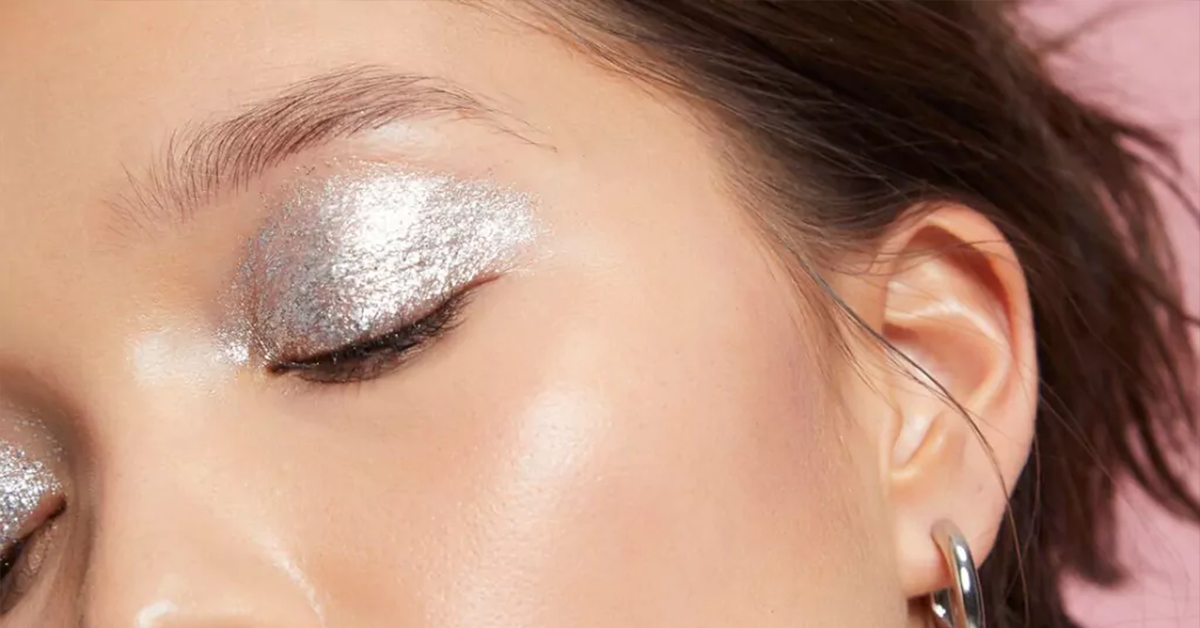This close-up image features a female model in a product photoshoot, likely for cosmetics. The photo is closely cropped, showcasing her eyes, part of her nose, ear, and long dark hair, which is tucked behind her ear and flowing towards a soft pink background. The model's eyes are closed to prominently display her bold, silver eyeshadow, complemented by mascara and foundation that highlight her smooth, clear skin. She wears a large, silver hoop earring that draws attention to her elegant look. The meticulous detailing of her makeup, especially the shimmering silver eyeshadow, suggests this image is intended for a makeup advertisement.